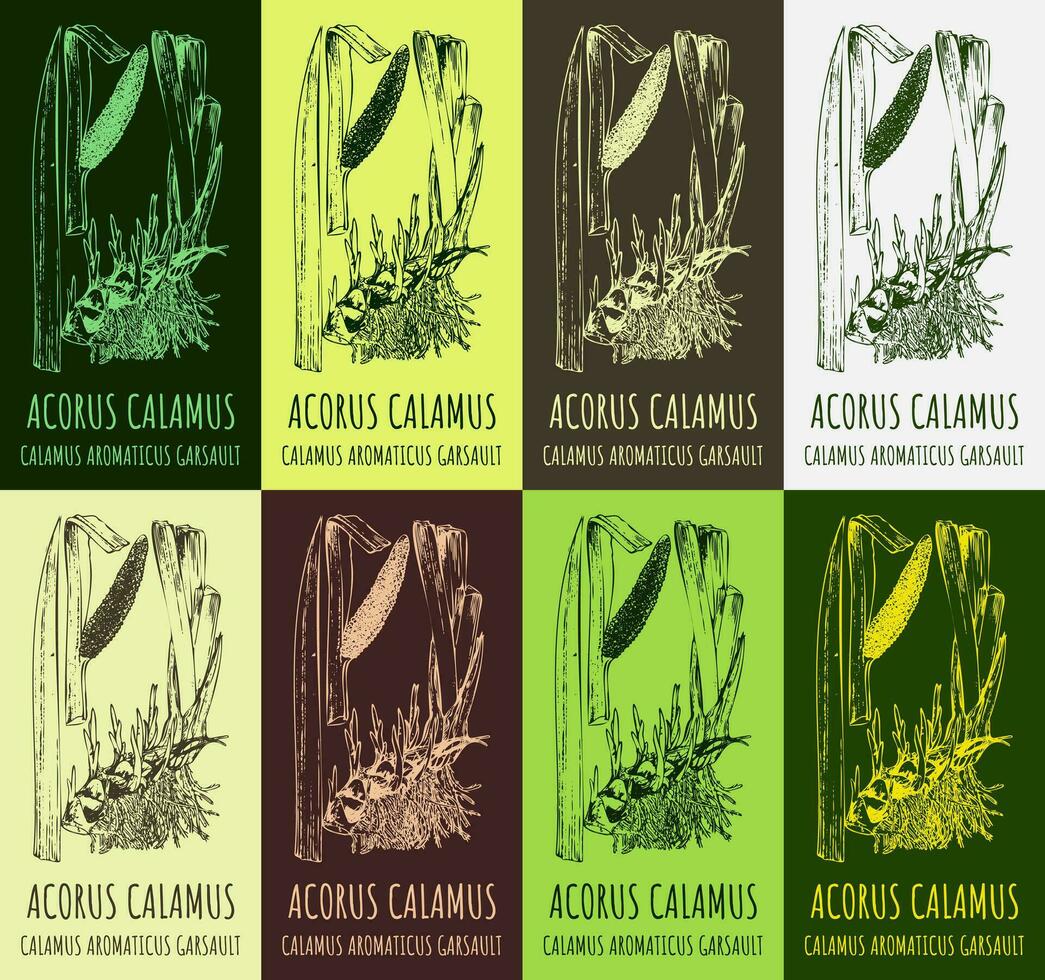The image features an eight-part diagram consisting of identical line art illustrations of the plant Acorus Calamus, also known as Calamus Aromaticus Garsault. Each illustration is presented against a different background color, which includes dark green, yellow-green, white, beige, dark brown, burgundy, bright green, and yellow. The drawings, resembling cattail plants with fuzzy tubular risers and folding leaves, are consistently labeled with "Acorus Calamus" at the top and "Calamus Aromaticus Garsault" at the base. The line art remains the same in each square, with only the background colors providing variation.